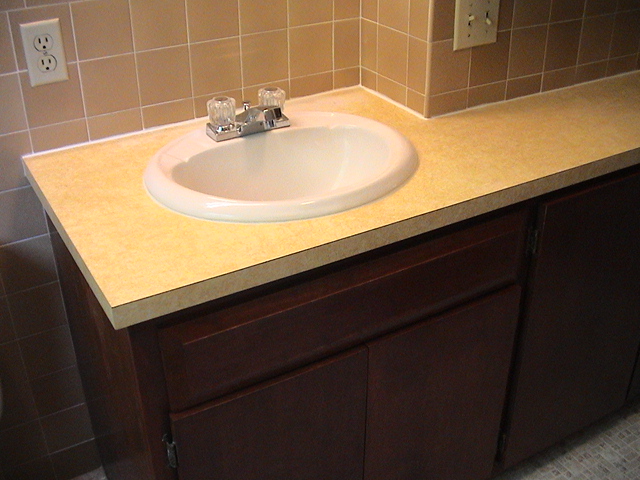A meticulously maintained sink, evocative of the 1970s or 1980s, sits prominently on a bathroom counter. The sink itself is a pristine white, oblong in shape, with a pair of silver spigots for hot and cold water. These spigots feature faux glass handles reminiscent of a bygone era. The countertop, a vintage yellow Formica about an inch thick, exhibits a subtle, consistent pattern rather than a solid hue. Beneath the countertop, the cabinets are simple and unadorned, finished in a dark brown with a false front panel and no visible hardware.

The backsplash is composed of square tiles in varying shades of light brown, meticulously grouted with white. On the left side of the backsplash, an off-white electrical outlet is embedded. The countertop extends thinner to the right of the sink, curving slightly, before meeting a light switch where the left toggle is in the "up" position and the right in the "down" position. The overall lighting suggests a source from above, casting the lower part of the photograph in shadow and leaving the cabinetry colors indistinct, while the sink and countertop remain brightly illuminated and in focus.